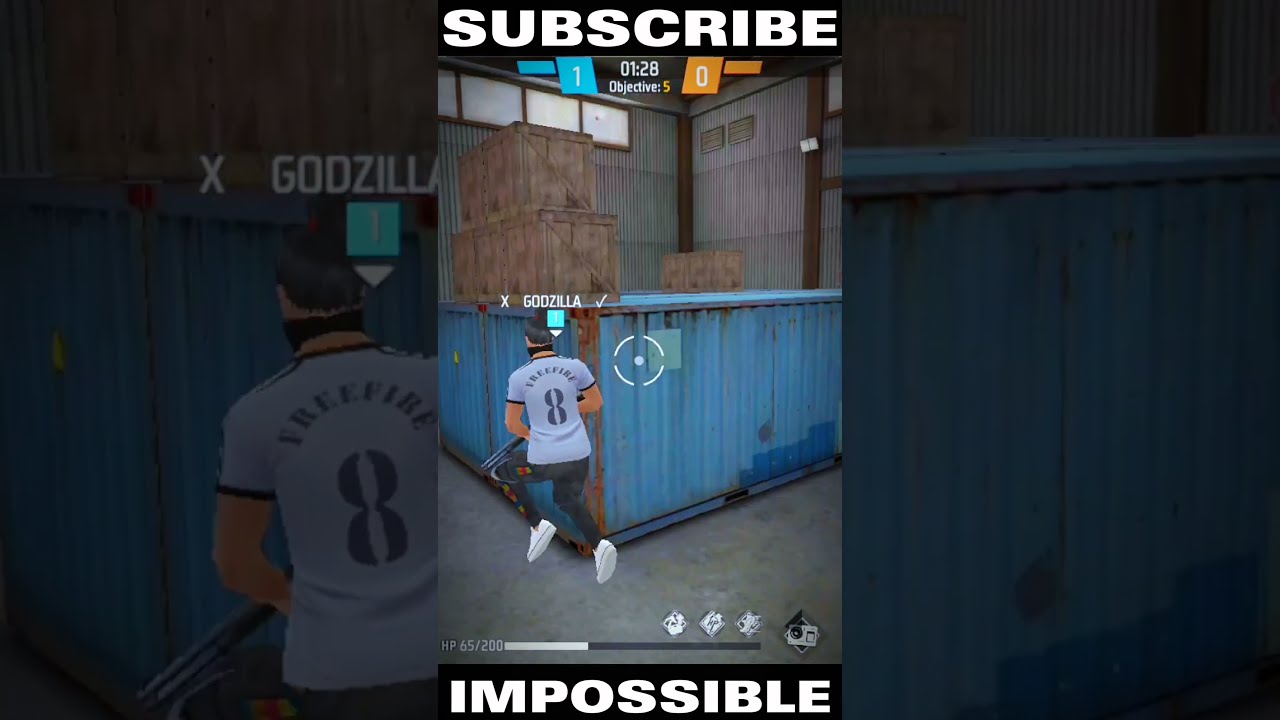A detailed screen capture from a shooter video game features a vertically oriented image of a character mid-action. Central to the scene is a light blue metal container, with wooden crates placed on top. To the left of center, a character sprints forward, back facing the viewer. The character is outfitted in a distinctive light gray shirt with dark blue lettering reading "Free Fire" at the top, and the number "8" below. Completing his outfit are blue jeans, white sneakers, a gray hat, and a black strap around his neck. His white sneakers are entirely off the ground, indicating dynamic movement. The top of the screen prominently displays the word "Subscribe" in bold letters. Just beneath this, a scoreboard shows "1" under a blue section on the left and "0" under an orange section on the right, along with a timer set at "01:28" and an objective indicator stating "5". At the bottom of the screen, the word "Impossible" is visibly centered above a progress bar reading "65 out of 200".